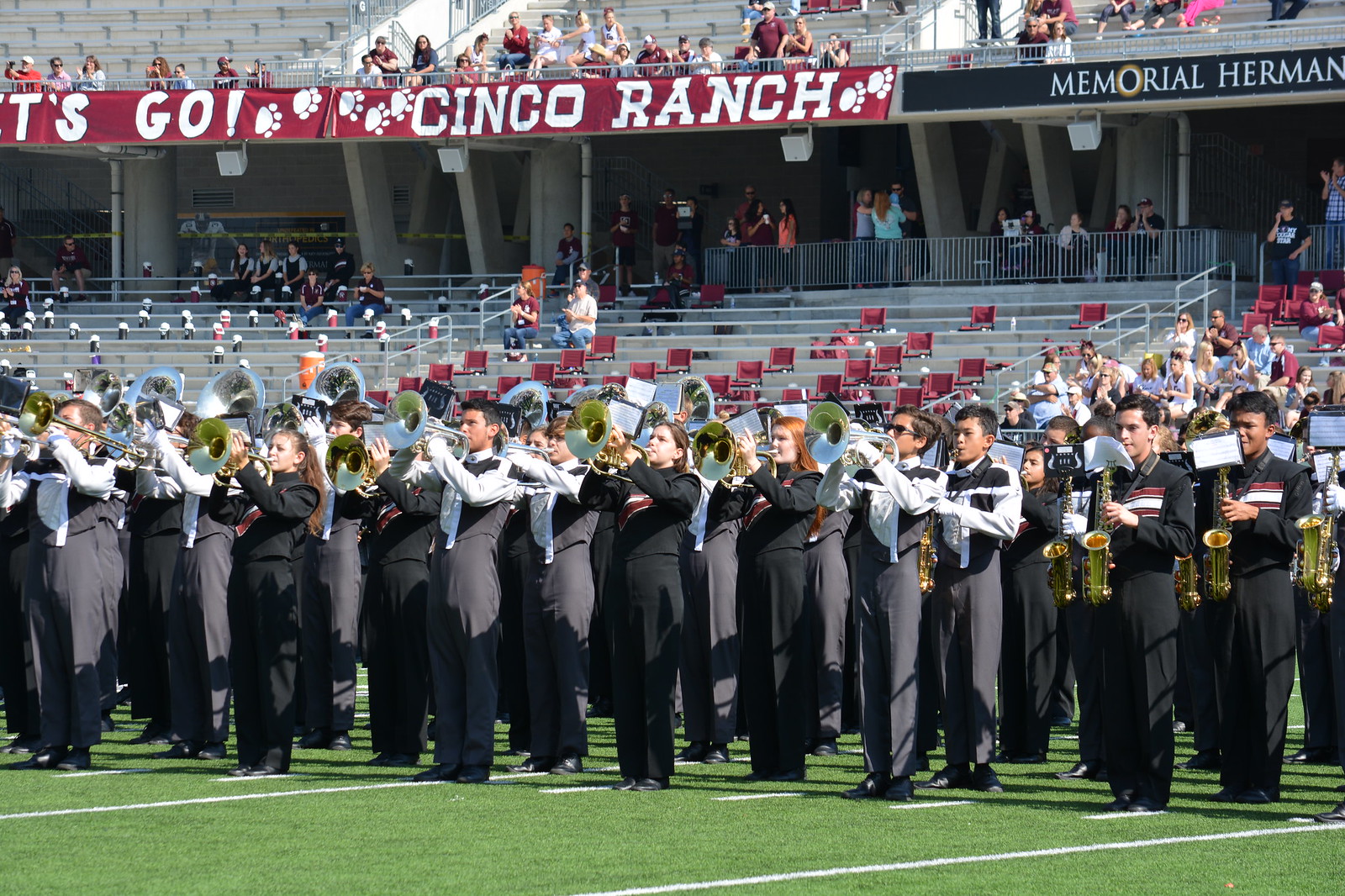The image captures a horizontally aligned rectangular picture of a marching band performing on a light green football field within a stadium. The band, situated towards the bottom of the image, occupies the full width from left to right. The musicians, facing slightly towards the left, are dressed in black pants and vests, some with long-sleeved white shirts, while others wear black tops. The instruments gleam gold and silver, and the front row on the right features saxophonists, while trombone players are positioned in the middle and left sections. White dashed and solid lines are visible on the field.

Behind the band, the lower level of stands is mostly empty, with a scattering of spectators wearing maroon and white shirts. The gray stands continue above, with maroon chairs and an additional row of seating at the top. A guardrail on the right and white railings frame the seating sections. Hanging from an overhang wall are banners and cream-colored speakers, while tables are positioned underneath the overhang. Prominent red and white banners with paw prints and text reading "Go Cinco Ranch! Memorial Hermann" adorn the top of the stands. The overall scene highlights the lively performance of the band amidst the stadium backdrop.